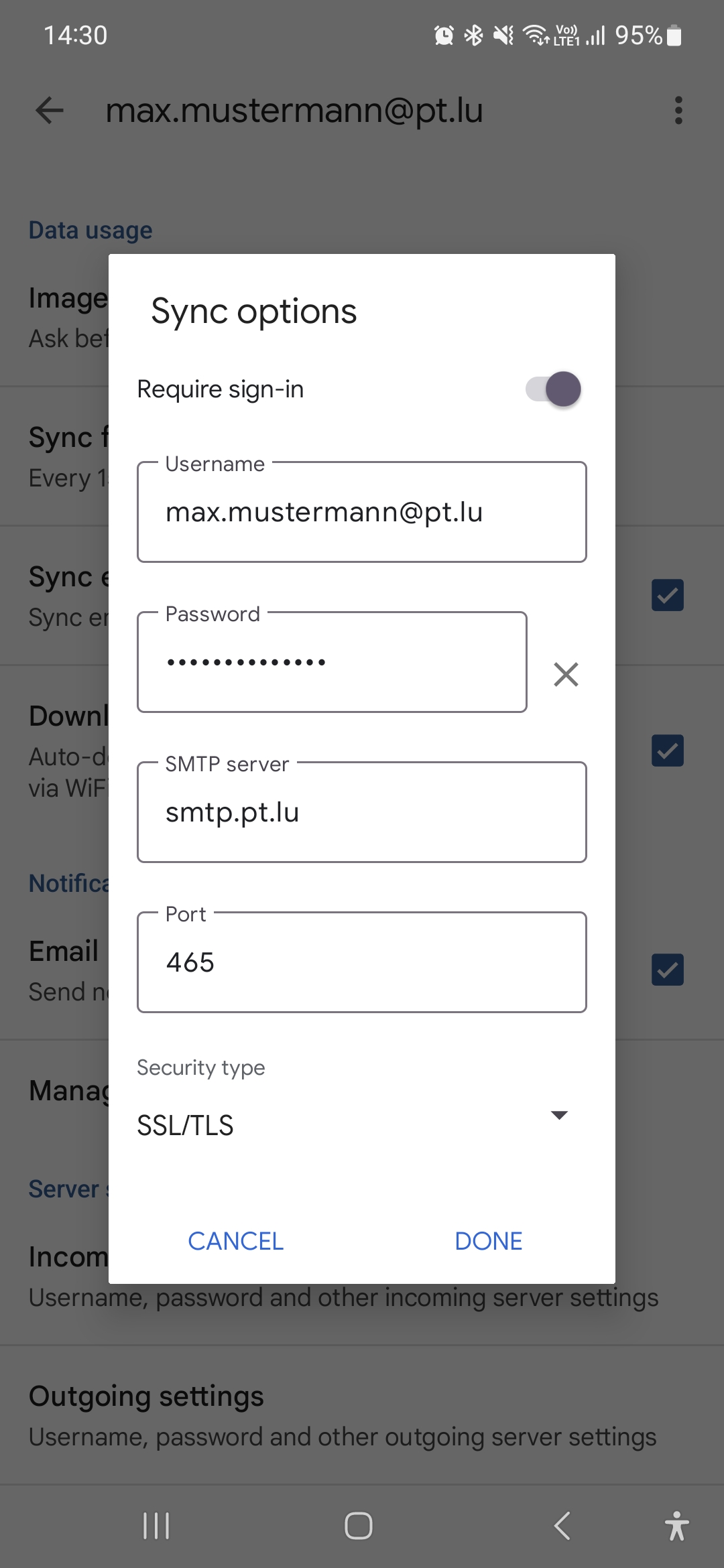The image depicts a screenshot of a phone displaying an open submenu superimposed on a preceding menu. The current submenu is labeled "Sync Options" and includes various fields and settings. One field, "Require Sign-In," is selected, revealing a username "max.musterman.pt.blue" and an associated password field. Below, there are settings for the SMTP server with details like "smtp.pt.blue" for the server, port number "465," and the security type "SSL-TLS." At the bottom of this submenu, "Cancel" and "Done" buttons are present.

The background reveals a previous menu, partially obscured but identifiable. It prominently displays the username "max.musterman.pt.blue" at the top along with a "Back" button. Sections partially visible in this background menu include "Data Usage," "Images," "Sync," and "Download," though exact details of these sections are hidden by the foreground submenu.

Additional elements confirm that this is a mobile phone screenshot. The top status bar shows the time as 14:30, a Wi-Fi signal, a Verizon LTE connection, and the battery level at 95%. The bottom of the screen features typical Android navigation buttons for home, back, and recent apps. This context supports the observation that the user is configuring synchronization settings on their device.